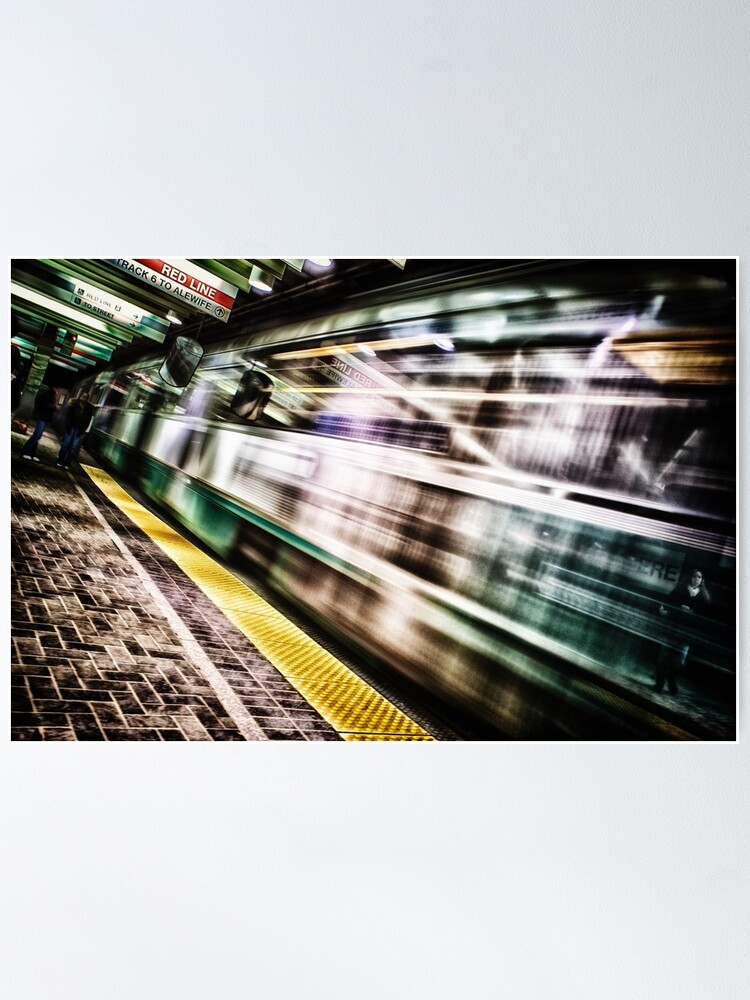This image features a dynamically edited underground subway scene framed by a gray border on the top and bottom. The central focus is a subway train in motion, with streaked lines in vibrant colors—white, green, blue, purple, and yellow—creating a sense of speed. A distinct yellow strip marks the edge of the platform, which is made of blackish and whitish bricks, emphasizing the station's gritty, urban feel. To the top left, a diagonal sign reads "Red Line, track to Alewife," with additional signs indicating train routes and stops visible in the background. The waiting area on the left shows a few people in jeans and dark jackets standing distantly. The entire scene captures the hectic energy and colorful blur of a bustling subway station.